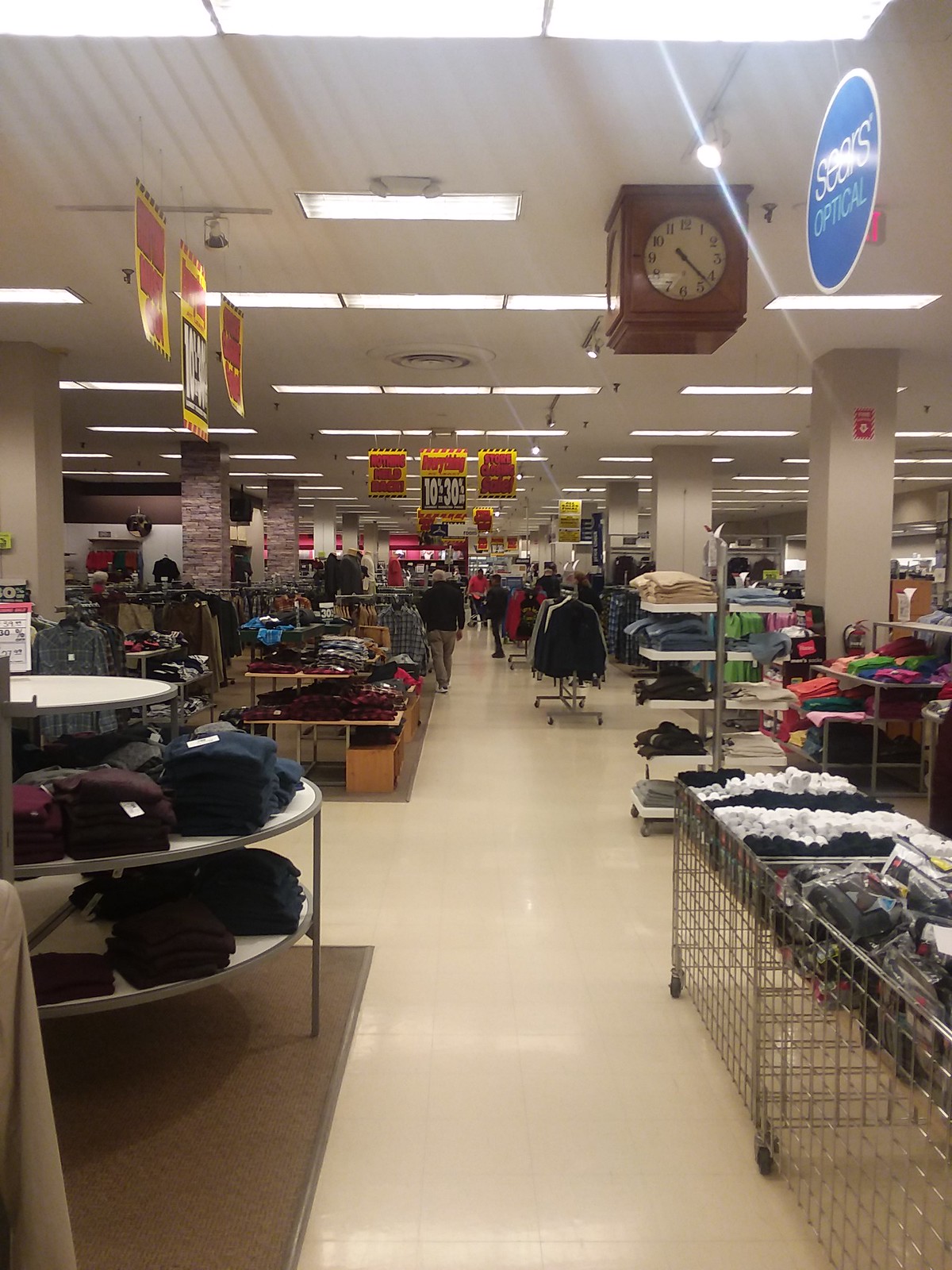The photograph captures the interior of a Sears department store, displayed in stark detail. Dominating the scene is a large, cube-shaped wooden clock suspended from the ceiling, with one clock face prominently visible and presumably faces on the other sides. The ceiling features white acoustic tiles interspersed with translucent plastic tiles housing fluorescent light fixtures, casting a bright yet artificial yellowish light over the scene.

Straight down the walkway, the store is divided into sections with off-white tile flooring and brown carpet. On the left side, circular shelving units hold neatly folded sweaters, while on the right, rolling wire carts are filled with socks. The cluttered aisles reveal various clothing racks and displays, showcasing a plethora of garments.

Prominent sale signs hang from the ceiling, emblazoned with yellow and red colors, announcing discounts of 10 to 30% off. A distinctive black box with white text also highlights the markdowns, hinting that the store might be undergoing a closure sale. The Sears Optical section is visibly marked by a blue sign. Despite a few people wandering through the store, the overall atmosphere feels empty and subdued, frozen in a specific moment in time.